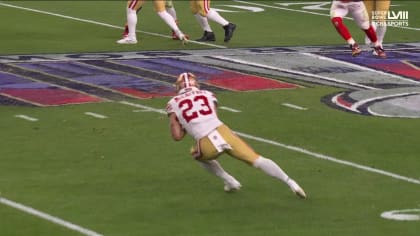The image is a still from an NFL football game featuring the San Francisco 49ers. Central to the composition is player number 23, who is in mid-action, rushing with the football held securely in both hands against his chest. He wears the 49ers' recognizable gold helmet adorned with a central white stripe flanked by red stripes. His uniform includes a white jersey displaying the red number 23, gold pants with distinctive red and white stripes down the sides, long white socks, and white football shoes taped around the ankles. The green grass field is marked with white yardage lines.

In the background, other players from the 49ers can be seen, partially visible and positioned predominantly in the upper middle and top right section of the image. A partially legible logo in the upper right corner suggests it is from the Super Bowl, displaying white text "LVI" and references to sports. This snapshot captures the intensity and style of a significant game, with colors prominently featuring gold, red, white, and hints of burgundy, green, purplish, and black.